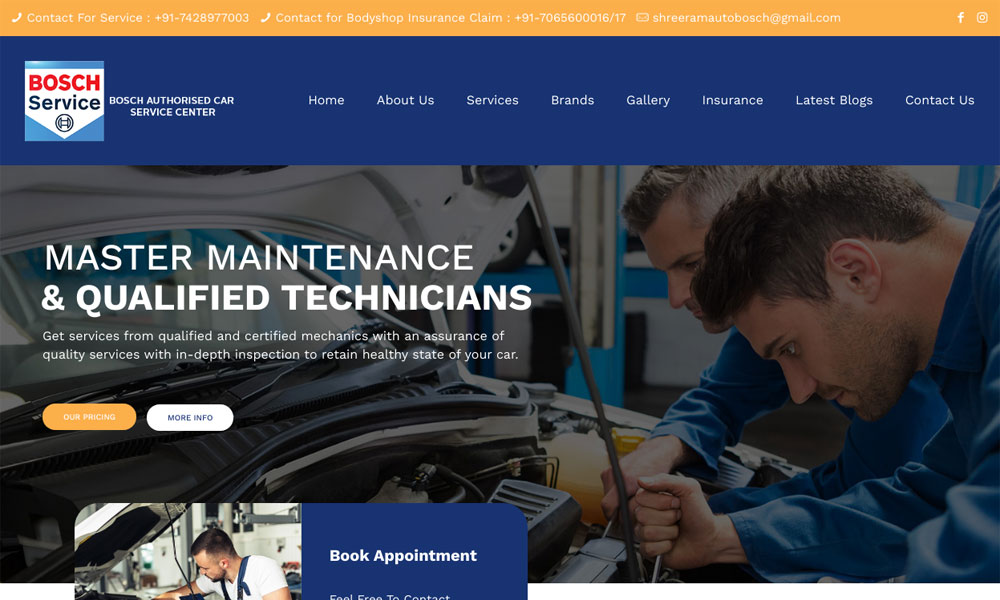"Welcome to BOTCH Services, the Authorized Car Service Center. An orange strip runs across the top, featuring contact information in white font: 'Contact for Service: 917-428-977003' and 'Contact for Body Shop Insurance Claim: 917-065-600061 / 17'. Also listed is the email for Sheeram (autobosh@gmail.com). On the right side of the strip, you'll find icons for Facebook and Instagram along with the BOTCH Services logo, which features a combination of blue, red, and white colors. Navigation options include Home, About Us, Services, Brands, Gallery, Insurance, Latest Blogs, and Contact Us. 

Below this header is an image of two mechanics diligently working on an engine. They are dressed in blue overalls and are Caucasian with short hair. To the left of the image, white text reads, 'Master Maintenance and Qualified Technicians.' The caption highlights that customers can expect service from qualified and certified mechanics, ensuring quality services with comprehensive inspections to maintain the health of their car. Below this text are two buttons: an orange button labeled 'Our Pricing' and a white button with dark blue text labeled 'More Info.'"